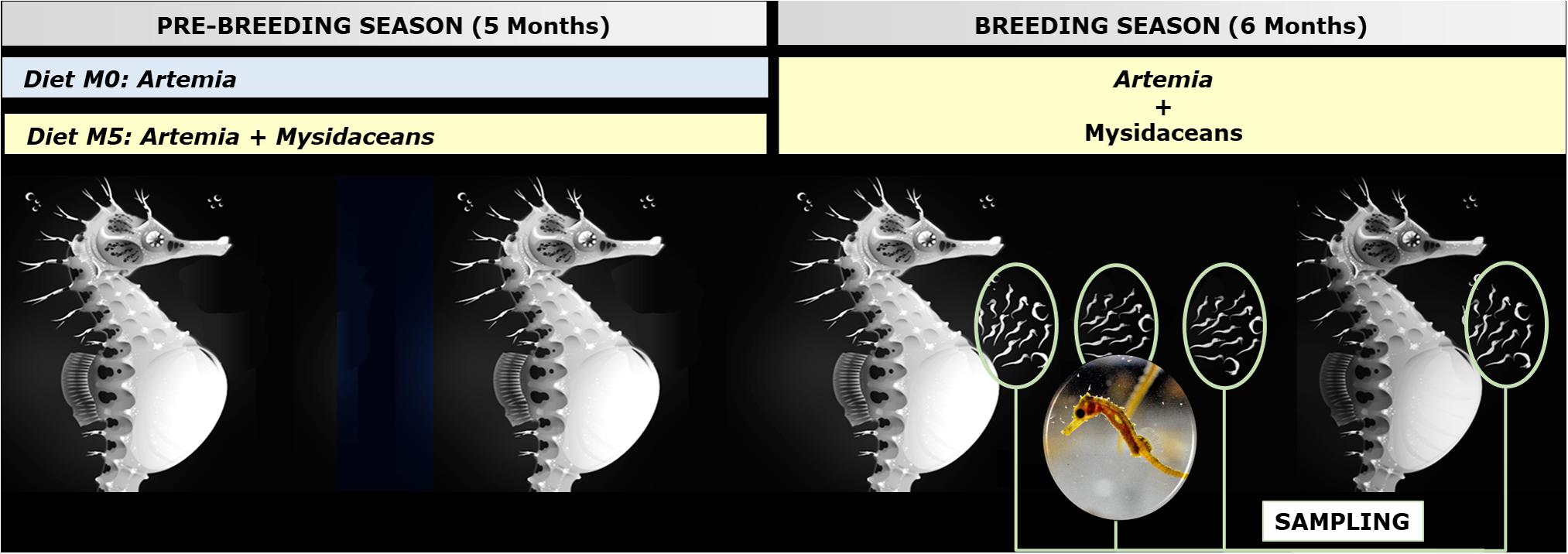This detailed caption integrates all the shared and repeated elements from the provided descriptions:

---

This image, in landscape view, features a detailed diagram depicting the breeding and dietary patterns of seahorses. The diagram is divided into two main sections: the left section, labeled "Pre-breeding Season (5 months)," and the right section, labeled "Breeding Season (6 months)." These sections highlight dietary intake: the pre-breeding diet includes M0 artemia, and M5 artemia plus mysidaceans; the breeding diet consists of artemia and mysidaceans. The bottom 60% of the image has a black background showcasing four white profile drawings of seahorses, all facing right. Notably, the two rightmost seahorses are accompanied by smaller seahorses emerging from their bodies. Between these two seahorses, there is a circle featuring a colored image of a seahorse. Below the seahorse furthest to the right, there is a label that reads "sampling." The entire slide has a yellow light tone and is notably wider than it is tall, with an aspect ratio approximately three times wider than tall.